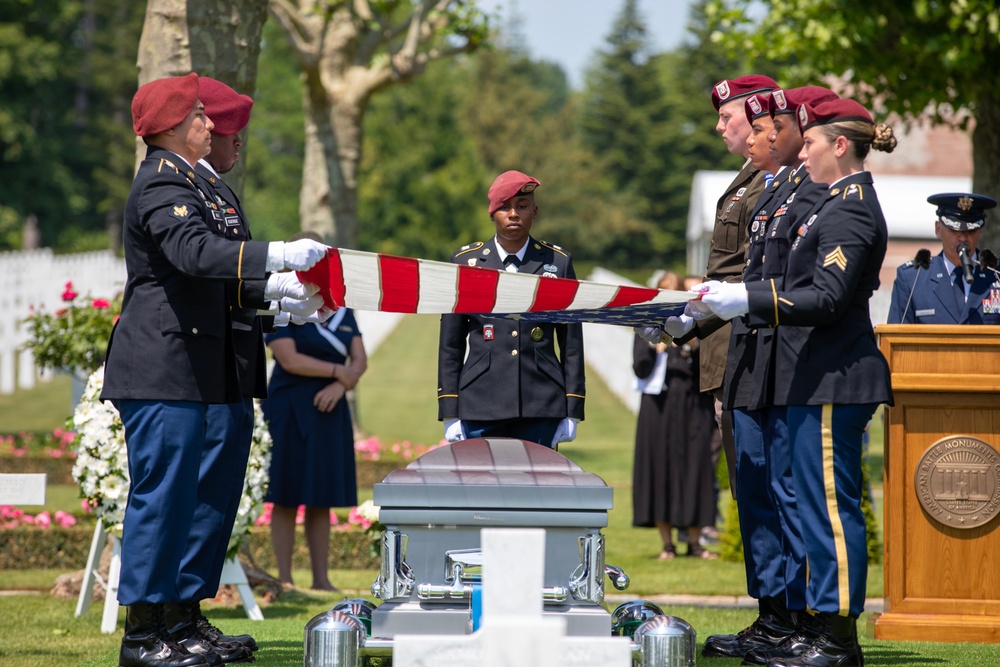In this poignant and solemn photograph of an outdoor military funeral, a silver metal casket occupies the bottom middle of the frame. Above the casket, two soldiers on the left and four on the right, dressed in dark blue jackets, light blue pants, black boots, and red berets, hold a stretched-out American flag. A white cross subtly obscures part of the casket. To the right, a uniformed military officer, outfitted in a blue jacket and blue hat, speaks into a microphone from a wooden podium, framed perfectly against the backdrop of tall, green trees, headstones, and funeral floral arrangements, all slightly blurred. Behind the casket stands another soldier, facing forward, seemingly ready to salute. In the distant background, the cemetery setting is further detailed with scattered grave markers and a hint of blooming flowers, while additional attendees, including some women in short blue dresses, are faintly visible. The scene captures the dignified and respectful atmosphere of a ceremonial farewell.